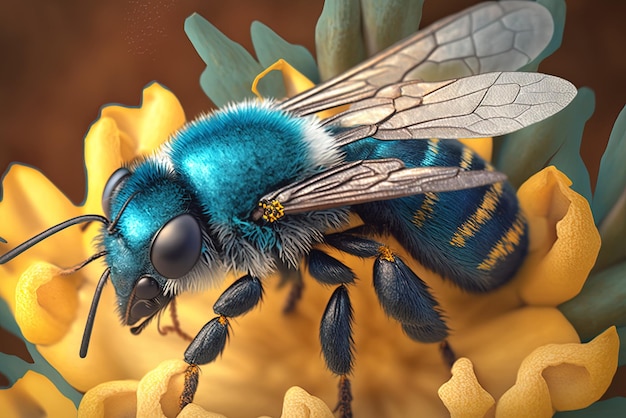This close-up image captures a striking turquoise blue bee, its fuzzy upper abdomen and head appearing blackish blue. The bee, with intricate translucent grayish-silver wings, perches on an open, blossomed yellow flower set against subtly reddish-hued background. Its black, hairy legs and black antennae, both dusted with pollen, are clearly visible. The bee's back abdomen displays vivid yellow stripes and its black eyes add to its detailed complexity as it actively gathers nectar and pollen. The flower itself is framed by green leaves, emphasizing the busy, strikingly colored bee in this detailed and vivid scene of pollination.